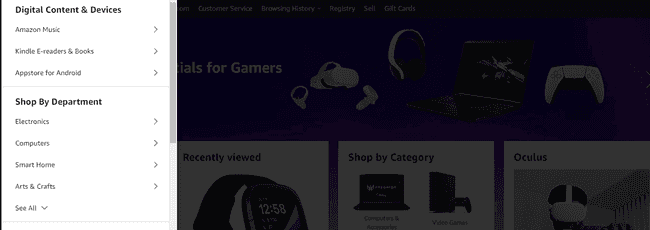This image is a screenshot of a webpage showcasing various electronics, primarily focusing on video game-related items. The webpage layout features several components, starting with a prominent blue header at the top, which includes a range of navigational images and promotional banners. The main section depicts an array of digital content and devices, such as laptops, gaming controllers, VR headsets like the Oculus, and other gaming accessories.

On the left side of the webpage, there is a detailed navigation menu presenting multiple categories for users to browse through, including Amazon Music, Kindle, Electronics, Computers, and Smart Home Devices. An 'All Categories' option is also available, allowing users to explore a comprehensive list of products beyond the highlighted selections.

Products are organized visually into different groups, with each category displaying related items. This structured presentation enables users to easily navigate through the different sections and find specific electronic products or digital content tailored to their interests.